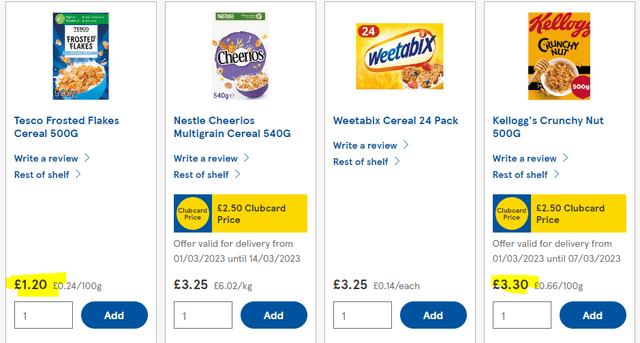This image depicts a web page listing breakfast cereals available for purchase. The page features four cereal options presented from left to right: Tesco Frosted Flakes, Nestlé Cheerios, Weetabix, and Kellogg's Crunchy Nut.

1. **Tesco Frosted Flakes Cereal (500g)**
   - Price: €1.20
   - Quantity: 1
   - Additional Options: Write a review, view the rest of the shelf.
   - Highlight: Price is marked in yellow.
   - Action: Add button available.

2. **Nestlé Cheerios Multi-Grain Cereal (540g)**
   - Standard Price: €3.25
   - Club Card Price: €2.50
   - Offer Validity: From 01/03/2023 to 14/03/2023.
   - Quantity: 1
   - Additional Options: Write a review, view the rest of the shelf.
   - Price Details: Includes both the cupboard price and discounted club card price.
   - Action: Add button available.

3. **Weetabix Cereal (24-pack)**
   - Price: €3.25
   - Quantity: 1
   - Additional Options: Write a review, view the rest of the shelf.
   - Action: Add button available.

4. **Kellogg's Crunchy Nut (500g)**
   - Standard Price: €3.30
   - Club Card Price: €2.50
   - Offer Validity: From 01/03/2023 to 07/03/2023.
   - Quantity: 1
   - Additional Options: Write a review, view the rest of the shelf.
   - Price Details: Includes both the regular and discounted club card price.
   - Action: Add button available.

Each cereal listing includes the option to write a review, view additional products in the respective categories, and add the item to the shopping cart through a prominently placed "Add" button. The prices are clearly indicated, with special offers and club card discounts highlighted and dated for customer convenience.